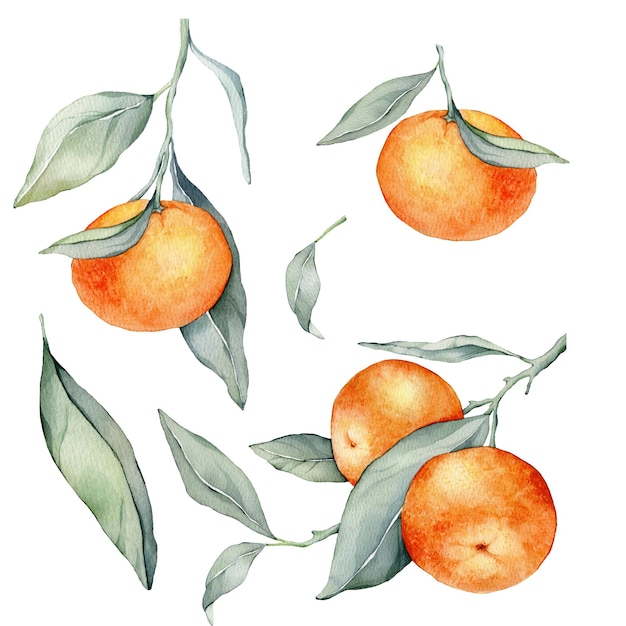This illustration from a book showcases a detailed watercolor painting of four oranges, which appear to be a type of citrus fruit, possibly unripe or exotic. The fruit is depicted on a branch, set against a white background. Each orange shows intricate shading, with lighter and darker orange areas that enhance their three-dimensional appearance. Accompanying the fruit are sage green leaves, some attached directly to stems, while a few float freely around the composition. Notably, one branch features two oranges side-by-side, separated by a leaf; another branch presents a single orange flanked by two leaves. Additionally, to the left of the image, an orange is framed by multiple leaves, with one large leaf prominently positioned behind it, and a smaller leaf in front. The arrangement includes loose leaves—a substantial one on the far left and a small, solitary leaf near the center—contributing to the overall aesthetic of the painting. This captivating illustration emphasizes both the beauty and the complexity of the depicted citrus fruit.